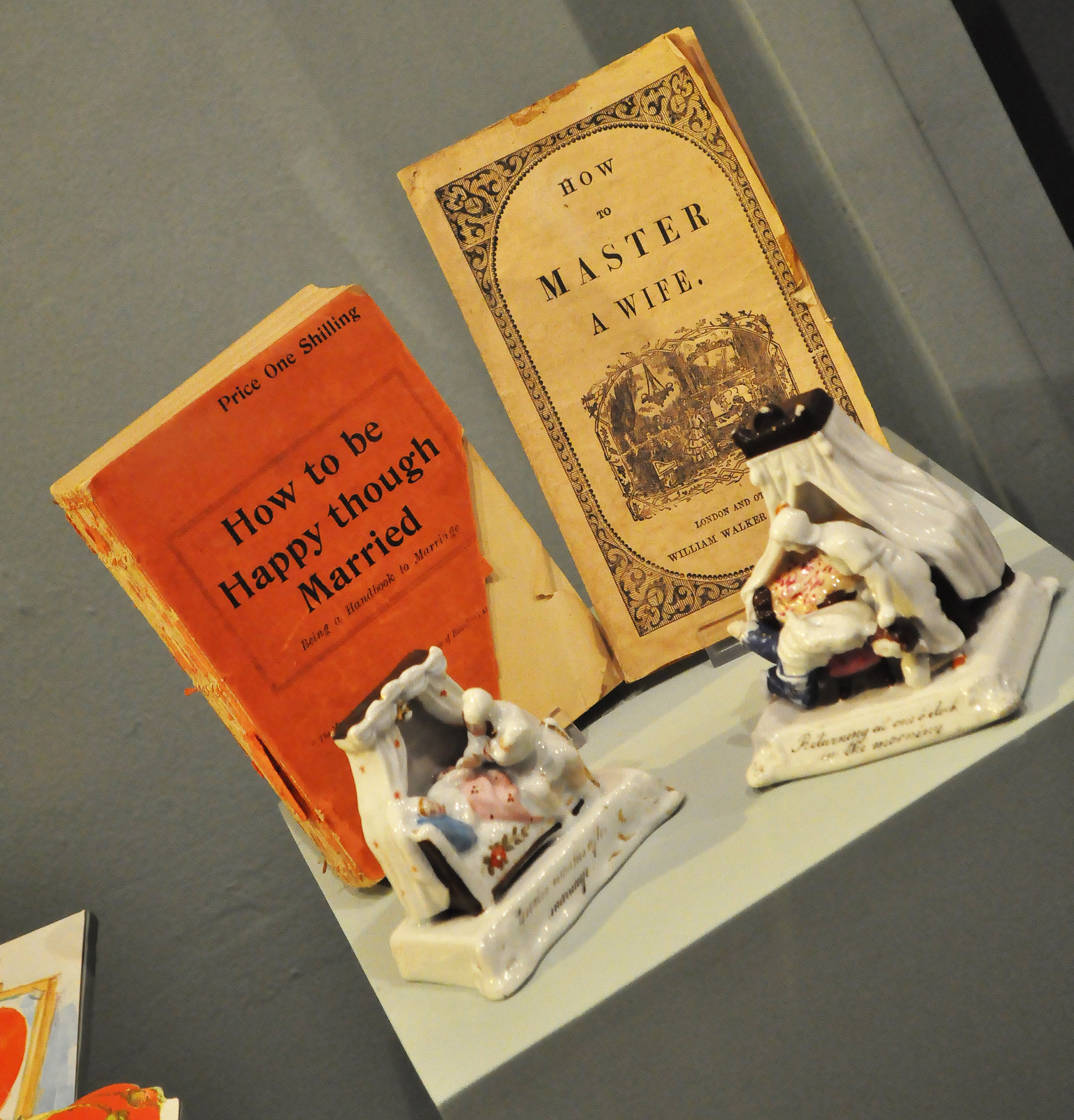Displayed against a dark gray background resembling a museum setting, the vertical rectangular image showcases two antique books positioned on a platform or pedestal. The book on the left, titled "How to be Happy Though Married," features a red cover with a yellow edge, though the bottom right corner is torn off, indicating its age and wear. The book on the right, "How to Master a Wife," has a yellow cover with brown printing and an illustration, along with a simple paper cover featuring a black ornate border. In front of each book stands a small, worn statue, with faded paint making their details hard to discern. The statues possibly depict significant historical or religious figures, with some suggesting they may represent baby Jesus, while another interpretation suggests a midwife scene. In the lower left corner of the image, a partial view of another display, likely another book, is visible.